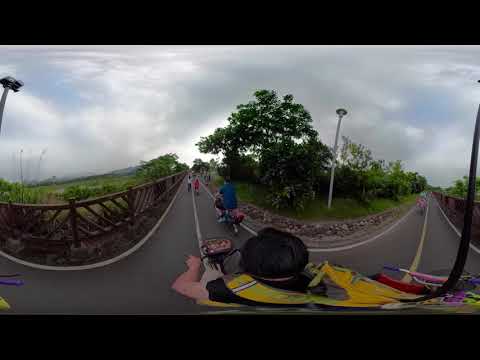The photograph captures an outdoor scene on a cloudy day featuring a group of cyclists navigating a narrow, two-lane road that resembles a bike path. In the immediate foreground, a person with black hair, wearing a yellow reflective vest over a black t-shirt, holds onto bicycle handlebars. The road appears distorted, likely due to a fisheye lens or panoramic mode, creating a W-like pattern towards the center of the frame. Ahead of the foreground cyclist, a man in a blue shirt is also riding a bike, and several more cyclists follow further down the path, though their specifics are blurred and grainy. On the left side of the road, there's a wooden fence, while the right side features a brick wall edging. Both sides are flanked by green grass, trees, and vegetation. The sky is partly cloudy with patches of blue and some gray clouds hinting at possible rain.